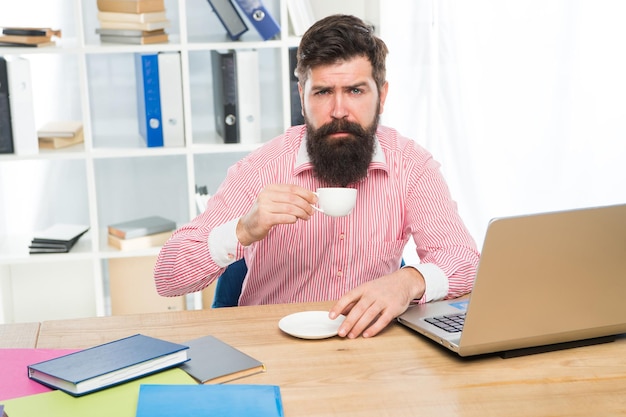The image depicts a man seated at a light brown, woodgrain-textured desk with books of various colors and sizes scattered across it. He is holding a small white cup, presumably of tea or coffee, with one hand over a matching white saucer. His other hand rests on the saucer. The man has a large brown beard, a mustache, and black hair that's longer on top and shorter on the sides. He is wearing a vertically striped pink (or reddish) and white collared button-down shirt with white cuffs. He appears to be frowning, looking directly at the camera, giving off a sad or distressed impression. In front of him is an open gray (or silver) laptop, suggesting an office setting. Behind him is a white bookshelf filled with various binders and other materials. A bright glow is visible to the right side of the image, hinting at a curtain bathed in natural light.